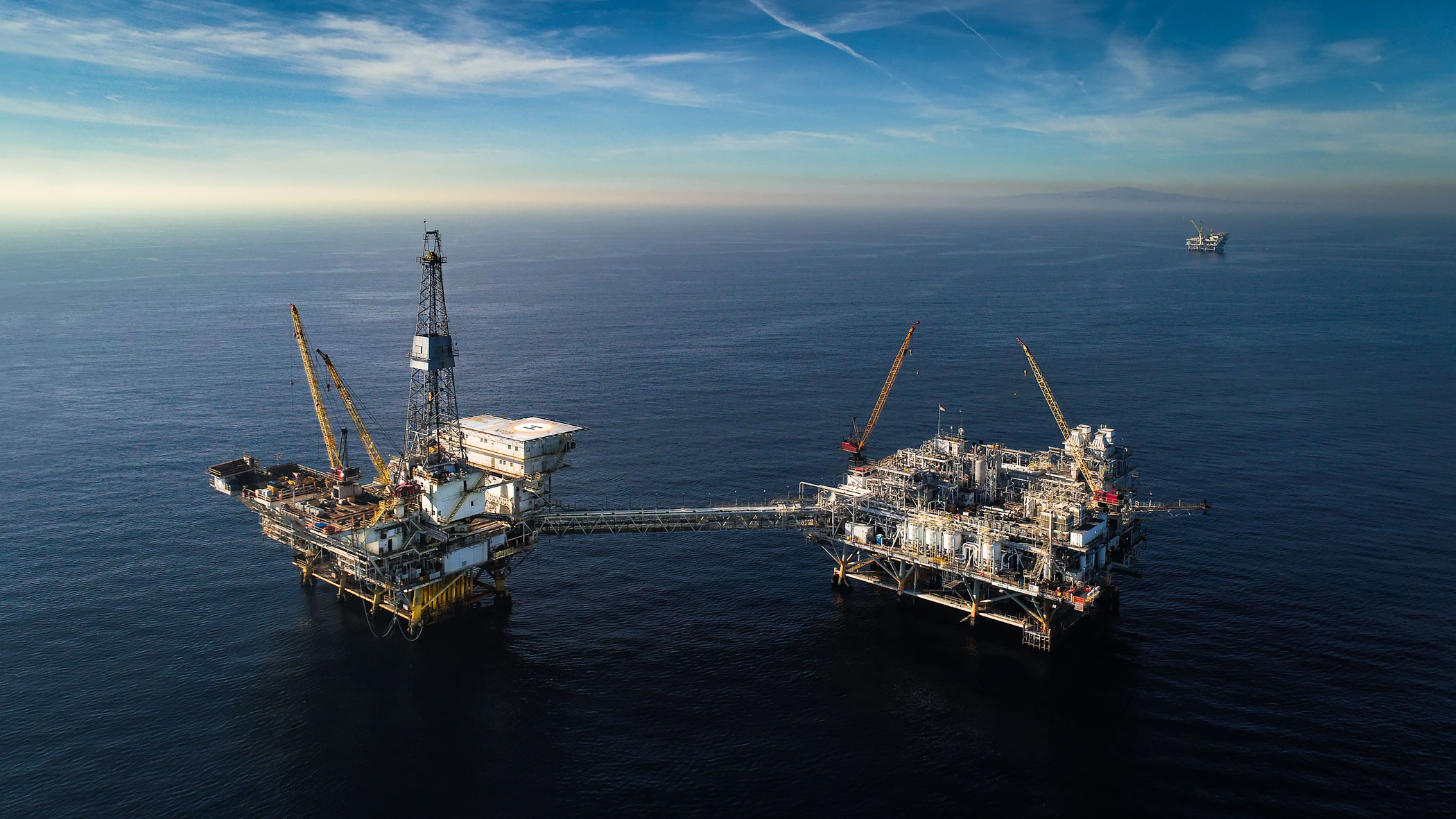The aerial photograph showcases two massive oil drilling platforms situated in the middle of a vast ocean, potentially the Gulf of Mexico. These platforms are interconnected by a bridge-like structure, possibly a conveyor belt or pipeline, signifying the transfer of resources between them. Each platform is equipped with two towering yellow cranes that extend high into the sky, emphasizing their mechanical dominance against the expansive blue backdrop. One platform also features a tall antenna tower and a helicopter pad, adding to its industrial complexity. Both structures are multi-story, with tanks and various construction equipment visible. In the distance, a large ship, likely an oil tanker, approaches, hinting at the ongoing extraction and transport of crude oil. The background features hazy mountains and a light fog, with another similar platform barely discernible on the horizon, beneath a sky dappled with white clouds shifting from light to darker shades of blue.